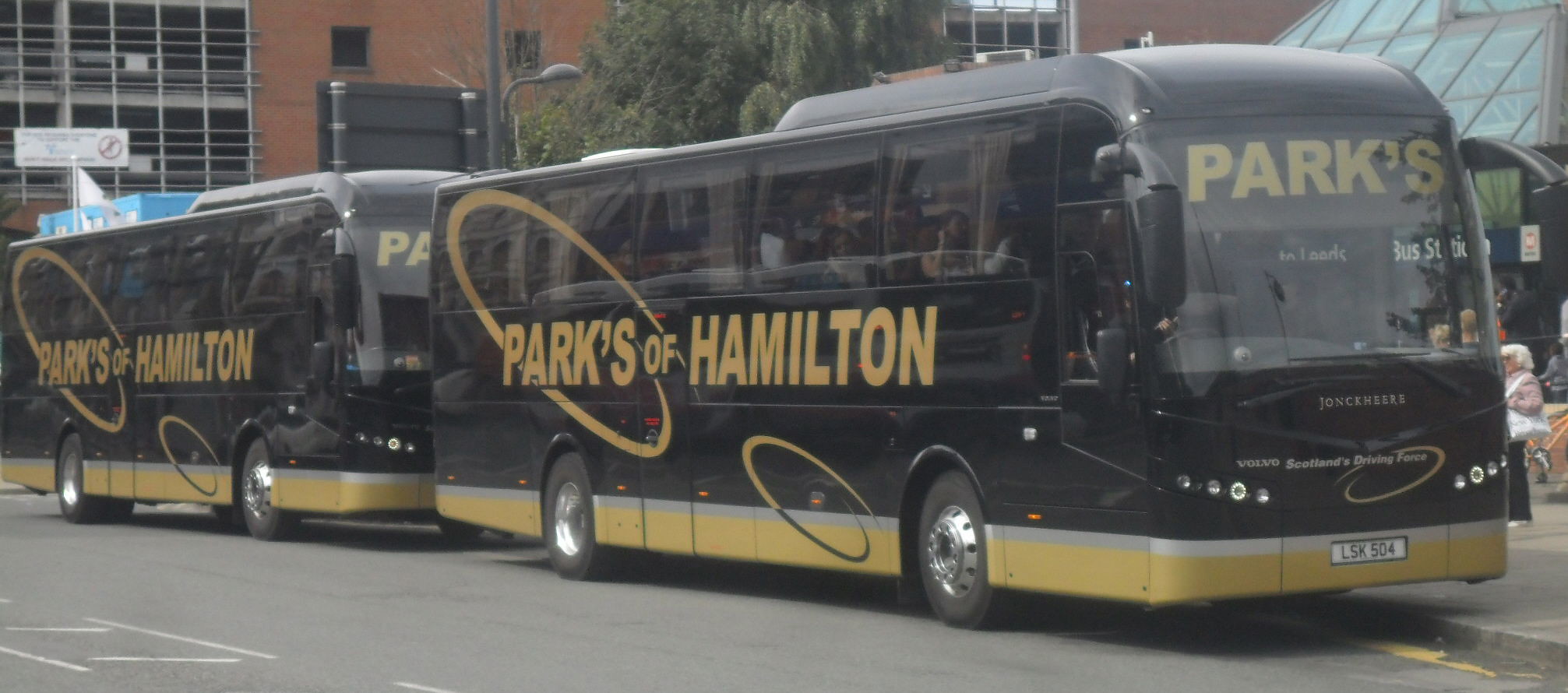In the photo, there are two large charter tour buses, both predominantly black with gold bottoms and gold text. The buses are positioned one in front of the other, each facing to the right. The text on the buses reads "Parks of Hamilton," with "Parks" emphasized by a large circle intersecting with "Hamilton." Additionally, "Parks" is prominently displayed on the front of each bus alongside the slogan "Scotland's Driving Force." The buses feature tinted windows, through which the outlines of passengers can be faintly discerned.

Behind the buses, a red brick building with black windows is visible on the left side, possibly a parking garage. A tree stands centrally between the buses in the background, with a glass-awninged building to the right. Underneath the awning, an elderly lady can be seen walking, and there are several people waiting near the far right bus. The day appears brightly lit, suggesting a sunny atmosphere.